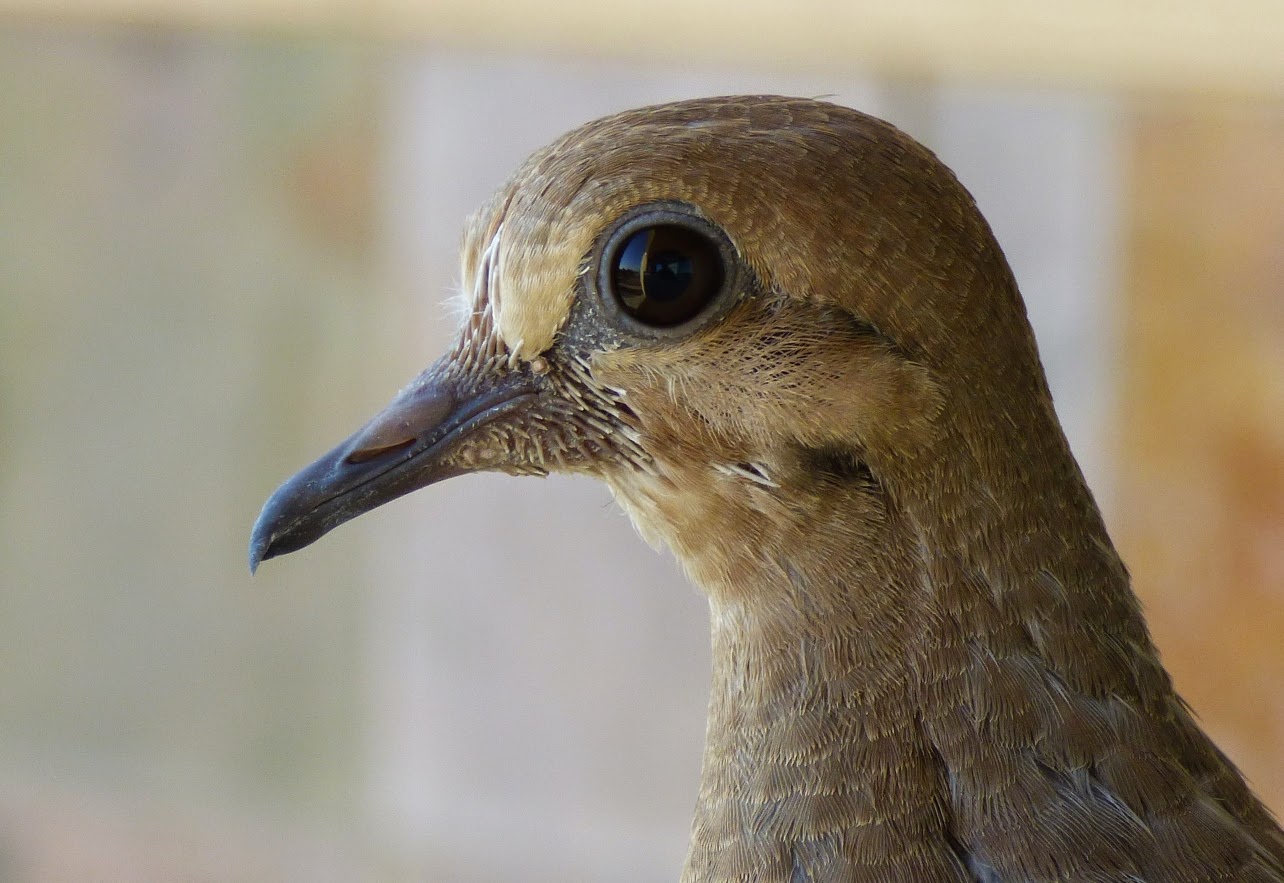This detailed close-up image features the head of a bird with strikingly large, black beady eyes. The bird has a pointed beak, primarily black or gray with a hint of brown atop, which suggests a prominent nasal structure. Its plumage consists of a pattern of light tan, dark brown, and brown feathers enveloping its head. The photo is significantly zoomed in, highlighting the bird's distinct facial features clearly.

Behind the bird, the background is out of focus but seems to showcase a white paper on a wall, indicating it is in a public place, likely just outside of a building. The reflected image of the person taking the photo is visible in the bird's eye, and one can discern the blue, cloudless sky captured in the reflection as well. Additionally, the shadow of the photographer appears near the bird. The bird is gazing towards the left side of the frame, and the indistinct building structure behind it further confirms that the setting is outdoors.